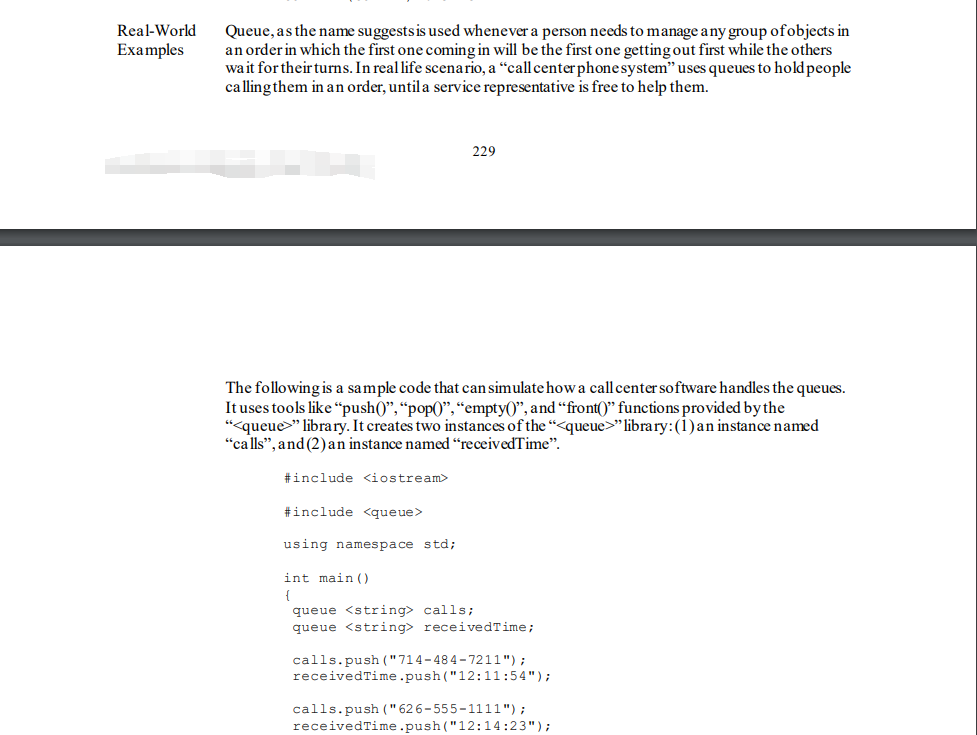In the realm of real-world applications, a Queue is a data structure that organizes elements in a First In, First Out (FIFO) manner. This organizational strategy is particularly useful in scenarios where order needs to be preserved, such as in a call center's phone system. In such a system, incoming callers are placed into a queue, ensuring that they are assisted in the order they arrived. This type of queue management enhances efficiency and fairness.

The provided example demonstrates how to simulate this type of queue management in a call center software using the 'queue' library. Key functions such as `push()`, `pop()`, `empty()`, and `front()` are utilized to manage the queue operations. The code snippet creates two instances from the queue library: one for handling the phone calls (`callQueue`), and one for tracking the time each call is received (`timeQueue`).

Below is an illustrated sample code outlining this process:
```python
import queue

# Create queue instances
callQueue = queue.Queue()
timeQueue = queue.Queue()

# Simulate incoming calls with timestamps
callQueue.put("714-484-7211")
timeQueue.put("121154")

callQueue.put("626-5511")
timeQueue.put("121423")
```

In this example, the `callQueue` holds the caller IDs (e.g., "714-484-7211"), while the `timeQueue` holds the corresponding timestamps when the call was received (e.g., "121154"). This structured approach allows the call center software to manage calls efficiently, strictly adhering to the FIFO principle to ensure that the first caller is the first one to be attended to.